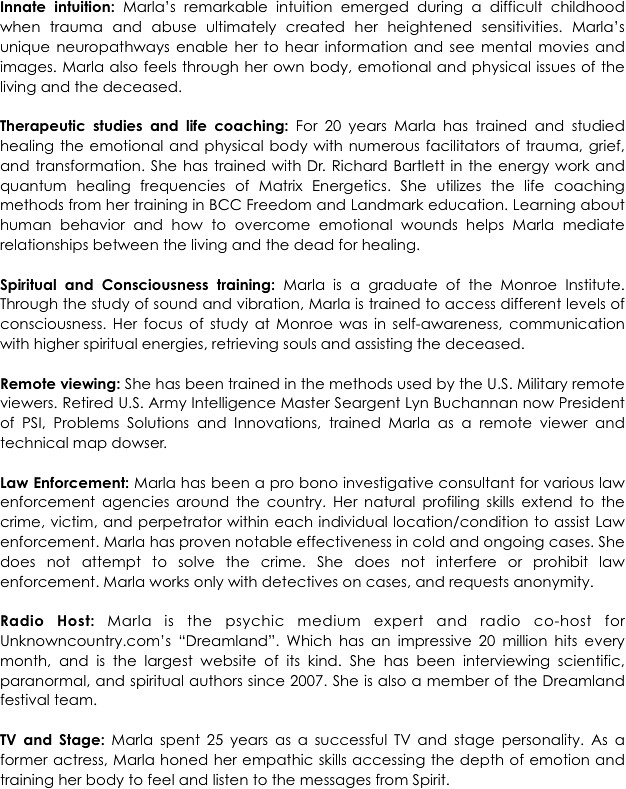This image consists of detailed black text on a white background, organized with headers and bullet points. The first section, titled "Innate Intuition," describes Marla's extraordinary sensitivity that developed from a traumatic childhood. Her unique neural pathways allow her to hear information and visualize mental movies and images. She can also sense emotional and physical issues in both the living and the deceased through her body.

The next section, "Therapeutic Studies and Life Coaching," outlines Marla's 20 years of experience in healing and the emotional, physical body. She trained with numerous facilitators in trauma, grief, and transformation, including Dr. Richard Bartlett, integrating energy work and quantum healing frequencies from Matrix Energetics. Using life coaching techniques from BCC Freedom and Landmark Education, Marla mediates relationships between the living and the dead for healing.

A third section, "Spiritual and Consciousness Training," highlights Marla's graduation from the Monroe Institute, where she studied sound, vibration, and different levels of consciousness. Her work involves moral and self-awareness, communication with higher spiritual energies, soul retrieval, and aiding the deceased.

Additional sections titled "Remote Viewing," "Law Enforcement," "Radio Host," and "TV and Stage" suggest further aspects of Marla's multifaceted career, although these paragraphs are not fully detailed in the provided text.